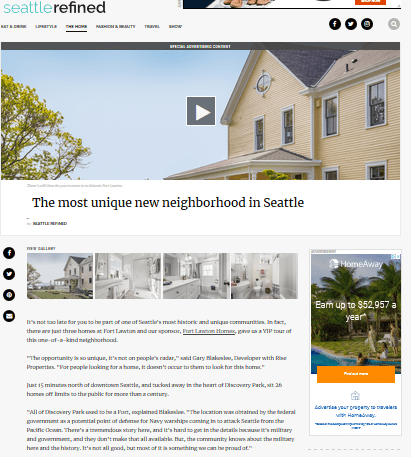This is a detailed caption for an image of the Seattle Refined website homepage:

---

The screenshot displays the homepage of the Seattle Refined website. At the top left corner, the website's name "Seattle Refined" is prominently featured, with "Seattle" in teal text and "Refined" in black. Below the title, there is a navigation bar with several tabs. Though somewhat difficult to read, it is clear that the "Home" tab is selected. To the left of "Home," there are tabs labeled "Lifestyle" and "Travel." On the far right, a tab appears to be labeled "Show," with more tabs in between that are hard to decipher.

Beneath the navigation bar, there is a large rectangular image capturing the upper portion of a house, including the top of the front facade and a portion of a tree to the left, set against a clear blue sky. A play button overlay suggests that this image is linked to a video. Below the image, a title reads, "The Most Unique New Neighborhood in Seattle."

Underneath the title, there are four smaller thumbnail images that appear to display various interior views of the house, providing a glimpse into its design and layout. Accompanying these images are three to four paragraphs of text, likely offering a detailed description of the house, although the small font size makes it challenging to read.

To the left side of the text, social media icons for Facebook, Twitter, Pinterest, and email are positioned for easy sharing. On the right side of the section, there is an advertisement featuring a tropical palm tree scene. The ad promotes home rentals with an earning potential of up to $52,957 annually. An orange button and small blue text are part of the advertisement, though the exact details are difficult to discern due to the small size of the text.